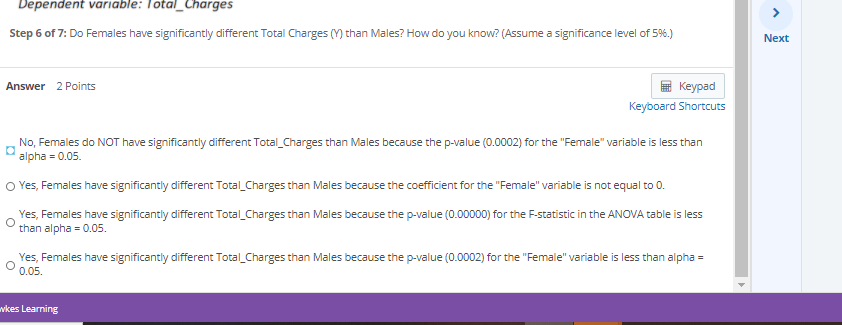The image is a horizontal rectangular graphic set against a clean, white background. The top edge of the image features black text partially cut off, reading "Dependent Variable: Total Charges." Below this text, spanning the width of the image, is a thin vertical rectangle with a scroll arrow at its base, adjacent to a light blue vertical area. To the right of this section is an icon: a bright blue greater-than sign enclosed within a shaded light blue circle, followed by the word "Next" in matching blue.

Directly below this, bold black text reads "Step 6 of 7:", followed by non-bold text stating "Do females have significantly different Total Charges (Y) than males? How do you know? (Assume a significance level of 5%)." A horizontal light gray line separates this text from the next section.

Next, in bold black font, the word "Answer" is followed by "2 points" in regular black font. On the far right, there's a white button labeled "Keypad" accompanied by an icon, and beneath it, medium blue text reads "Keyboard Shortcuts."

Returning to the main text, the answer provided is: "No, females do NOT have significantly different Total_Chargs than males because the p-value (0.0002) for the 'Female' variable is less than Alpha = 0.05." To the left of this text is a small box bordered in turquoise.

Below, three statements, each prefixed by an unfilled circle, provide alternative answer choices:
1. "Yes, females have significantly different Total_Chargs than males because the coefficient for the 'Female' variable is not equal to zero."
2. "Yes, females have significantly different Total_Chargs than males because the p-value (0.00000) for the F-Statistic in the ANOVA table is less than alpha = 0.05."
3. "Yes, females have significantly different Total_Chargs than males because the p-value (0.0002) for the 'Female' variable is less than alpha = 0.05."

At the bottom, a purple rectangular area contains text in white font. The first word is cut off on the left-hand edge, but "Learning" is fully visible.